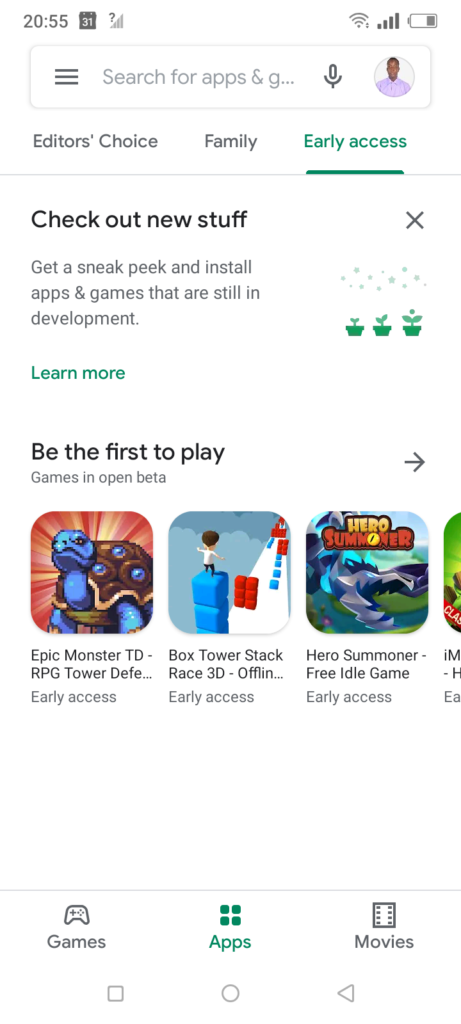The image showcases a screenshot of a smartphone interface, prominently featuring its status bar at the top. In the upper left corner, the time is displayed as 20:55, next to a counter showing the number "31" and an icon resembling a Wi-Fi signal with a question mark beside it. This icon is not immediately recognizable, potentially indicating an issue with the Wi-Fi connection. Moving to the right, standard icons for Wi-Fi, cell signal strength, and battery level are visible.

Below the status bar, a user interface element with three parallel lines suggests a menu option. Next to it, there is a search field accompanied by a microphone icon on the right side, allowing for voice search. An avatar icon, likely representing the user's account, is also present.

Further down, there are three menu tabs: "Editor's Choice," "Family," and "Early Access," with the latter highlighted in green, indicating it is currently selected. A heading beneath this section reads, "Check out new stuff," with a close button ("X") on the far right side to dismiss the message.

The section under the heading provides a brief description, "Get a sneak peek and install apps and games that are still in development," followed by a "Learn more" link in green.

To the right, there are three icons resembling potted plants, possibly with raindrops over them, though the representation is unclear. Below this section, there is a prompt, "Be the first to play," followed by "Games in open beta" and an arrow pointing right. Finally, at the bottom, three tiles display different games currently available for selection and open beta testing.